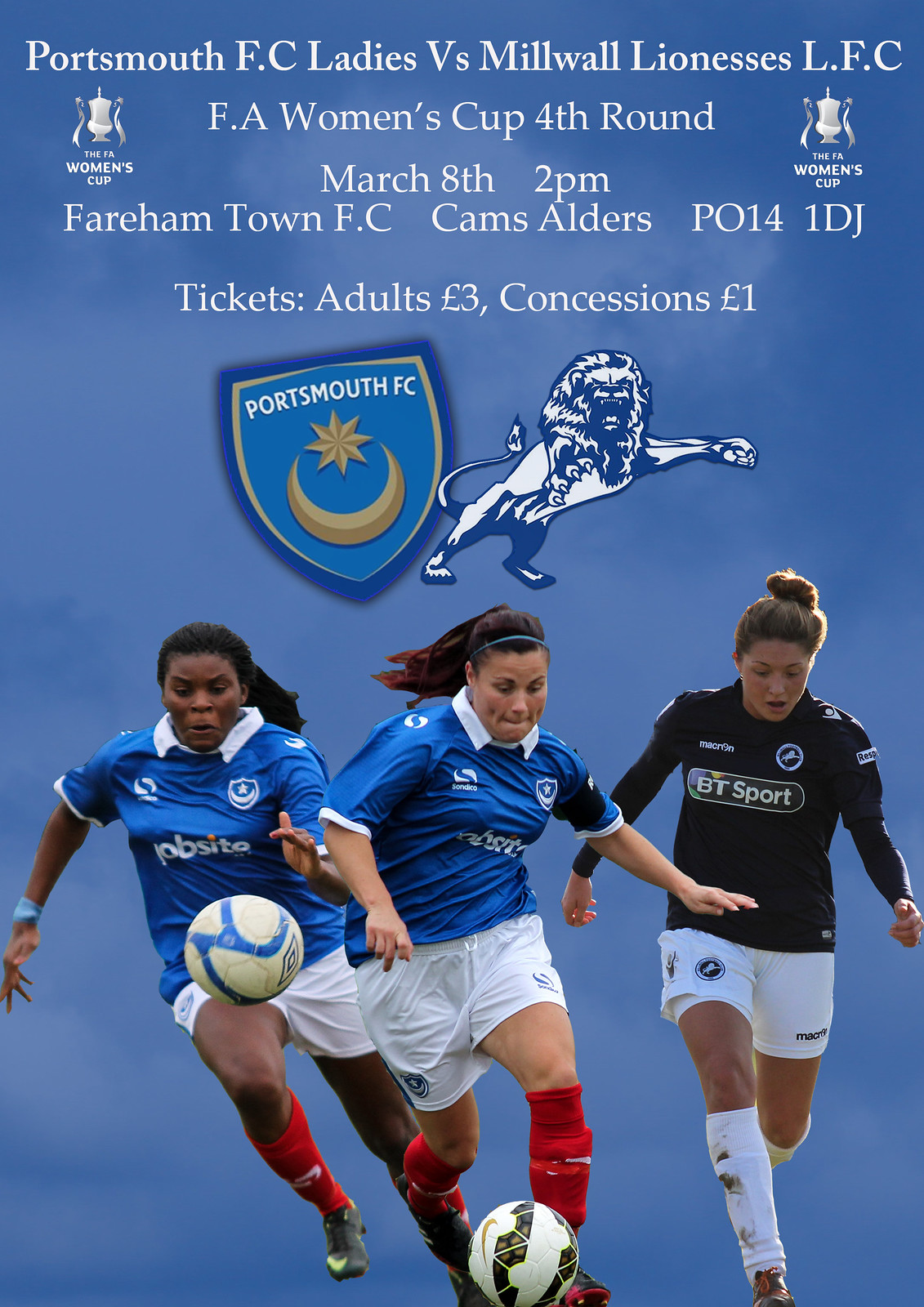The image advertises an upcoming FA Women's Cup 4th Round soccer match between Portsmouth FC Ladies and Millwall Lionesses LFC, scheduled for March 8th at 2 PM at Fairham Town FC, Cam Alders, PO14 1DJ. Tickets are priced at £3 for adults and £1 for concessions. The top of the image features white text on a blue sky background, reading "Portsmouth FC Ladies vs. Millwall Lionesses LFC, FA Women's Cup 4th Round, March 8th, 2 PM, Fairham Town FC, Cam Alders, PO14 1DJ, Tickets: Adults £3, Concessions £1." Below the text are logos of Portsmouth FC, including a blue shield with a moon and a sun, and a blue and white lion. At the bottom of the image are three female soccer players: the leftmost player, a black woman, in a blue jersey with "Job Site" on the front, white shorts, red socks, and black cleats, is running forward with a soccer ball near her knees. The middle player, a young white girl in the same blue jersey, white shorts, and red socks, is kicking a ball. The rightmost player, another young white girl, wears a black top, white shorts, and white socks. The players are set against a blue sky background, enhancing the overall energetic and inviting atmosphere of the advertisement.